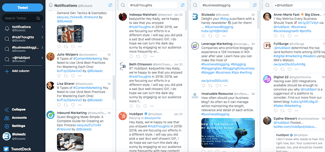This is a small, somewhat blurry screenshot of an older Twitter interface, distinctly different from the current "X" platform. The image displays several posts, including retweets and shares, although the details of the posts are unclear due to the image's size and quality. The left side of the interface shows a notifications tab, while the tweets appear on a white background, a feature characteristic of Twitter's earlier design. The interface itself is in a dark color scheme, either black or navy blue, and includes a prominent blue tweet button, which may no longer be present in the latest versions of the platform.